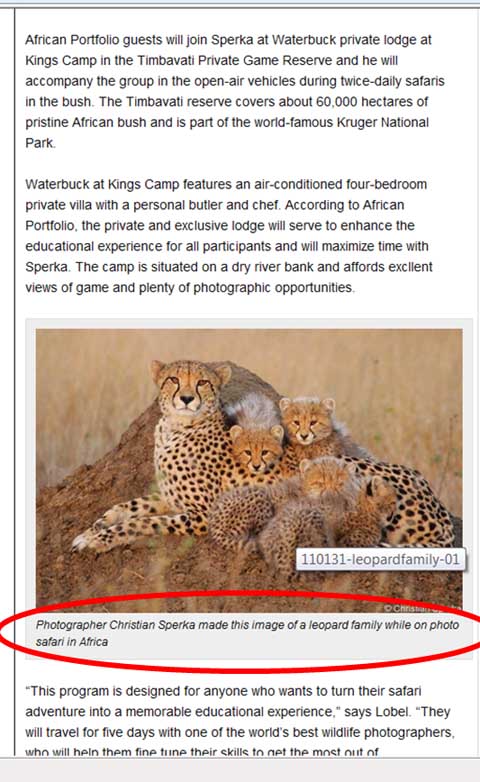The image is a screenshot of a Wikipedia page, although no title is visible, suggesting the page has been scrolled down. The top part of the screenshot features a block of text, and the bottom part contains additional text, surrounding a large central image. The image displays a leopard family and is labeled "110131-LeopardFamily." The caption, which is conspicuously circled in red using an editing tool, reads: "Photographer Christian Sperka made this image of a leopard family while on photo safari in Africa."

The text in the article provides detailed context about the photograph and Christian Sperka's work. It mentions that guests staying at Waterbuck Private Lodge—a location featured on Sperka's website, African Portfolio—can join him for safari photo opportunities. This indicates that the image serves not only to showcase the beauty of the leopard family but also to promote a unique business endeavor where guests can book stays and participate in photographic safaris led by Sperka himself.